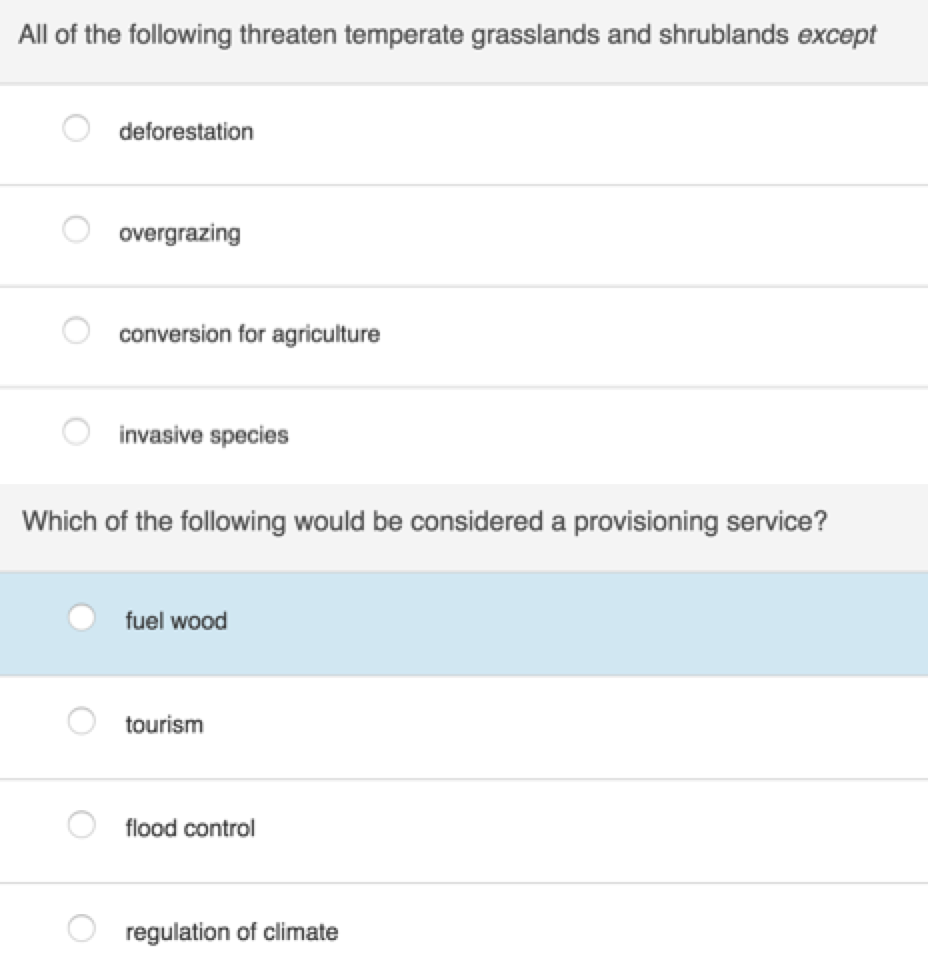The image showcases a section of a website designed for educational purposes, featuring a thin gray header spanning the top. In this header, a question is prominently displayed: "All of the following threaten temperate grasslands and shrublands except." Below this question, a multiple-choice format is used, presenting four possible answers, each accompanied by a hollow circular checkbox. The answer options are:

1. Deforestation
2. Overgrazing
3. Conversion for agriculture
4. Invasive species

Further down the page, a second question is posed within another gray section: "Which of the following would be considered a provisioning service?" Four options are listed here as well, with hollow circular checkboxes to the left of each answer:

1. Fuel wood
2. Tourism
3. Flood control
4. Regulation of climate

Notably, the entire panel for the first option, "Fuel wood," is highlighted in blue, suggesting it has been selected or emphasized in some manner. The layout implies it could be either part of an exam or study material, but this context is not explicitly provided. The clean design and structured format suggest ease of use for educational assessment or review.